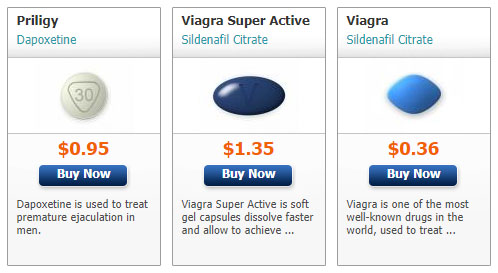This image is a detailed screenshot structured as a card detailing descriptions of medications across three columns. Each column provides information about a specific medication, including its name, active ingredients, visual appearance, and pricing, accompanied by a "Buy Now" button.

In the first column, the medication is depicted with the following details:
- The header reads "Priligy" in bold black text.
- Below it, in blue text, is "Dapoxetine."
- An image of the medication shows a white pill with "30" inscribed within a triangle.
- Underneath the image, the price is stated as $0.95, written in orange.
- A blue "Buy Now" button is positioned beneath the price.
- Priligy (Dapoxetine) is described as used for treating premature ejaculation in men.

The second column features:
- "Viagra Super Active" as the title.
- The active ingredient, "Sildenafil Citrate," is noted.
- The image displays a blue pill.
- The cost per pill is indicated as $1.35.
- Below the price is a blue "Buy Now" button.
- Viagra Super Active is characterized as soft gel capsules that dissolve faster, aiding in the timely achievement of desired effects.

In the third column, the details are about:
- "Viagra" (standard version).
- It also contains "Sildenafil Citrate."
- The pill is shown as a blue diamond shape.
- The pricing is set at $0.36 per pill.
- A "Buy Now" button in blue is present below the price.
- Viagra is recognized as one of the most well-known medications worldwide, primarily used to treat erectile dysfunction in men.

Overall, this screenshot provides a detailed, comparative overview of these medications, including visual elements, pricing, and their intended uses.